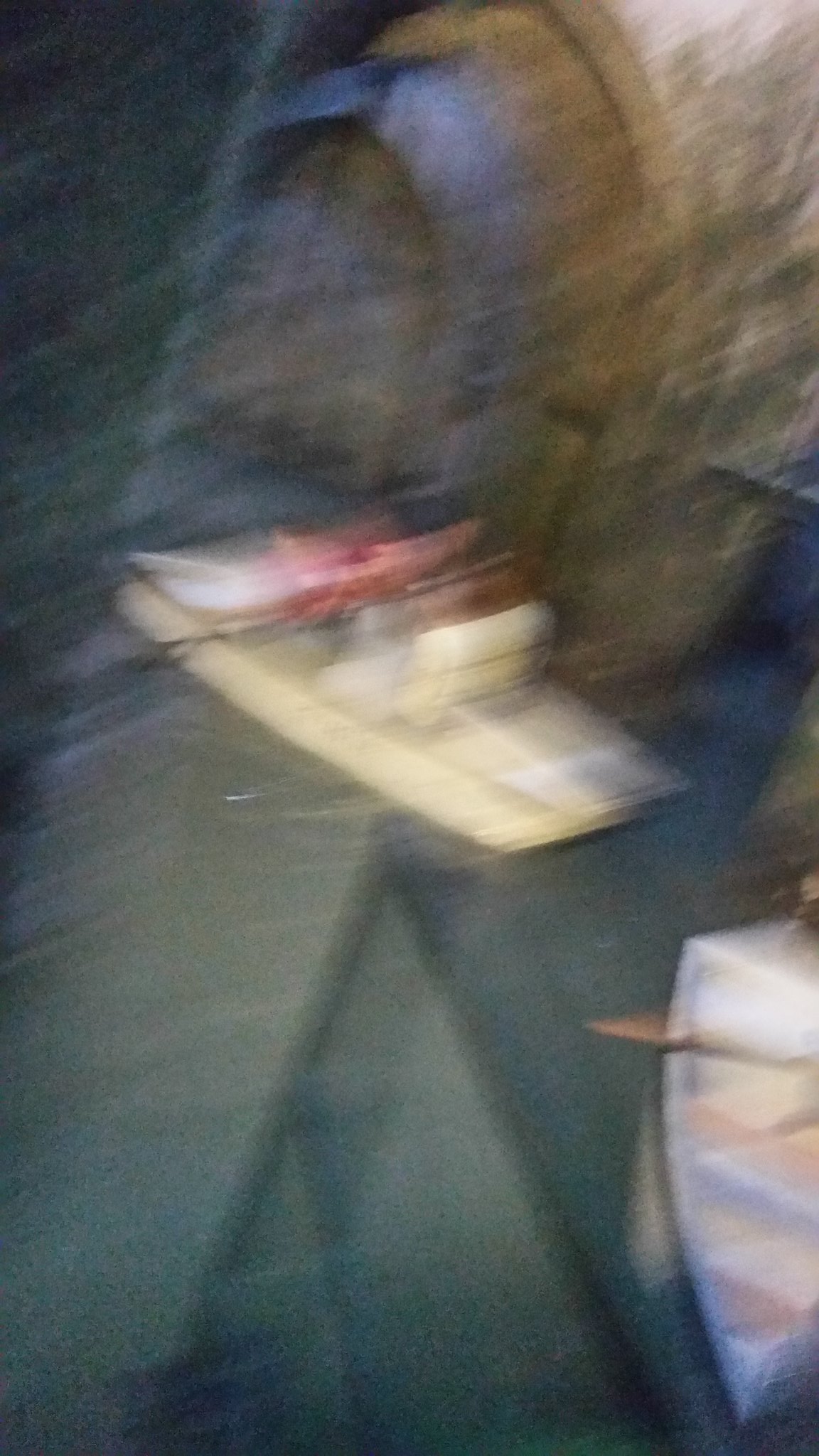In this very blurry image, the scene appears to be set in an amusement park, specifically depicting a ride that involves small, themed boats navigating through a haunted house attraction. Although the visibility is poor, two distinct boats can be identified traveling near a weathered wooden structure with a shallow open entrance. One of the boats is more squared and painted yellow, while the other features a pointed, multicolored front and a predominantly white rear. The oars attached to these boats suggest a manual or guided waterway experience. The detailed textures of the wooden structure and the boats lend to the eerie, antiquated atmosphere typical of haunted attractions.